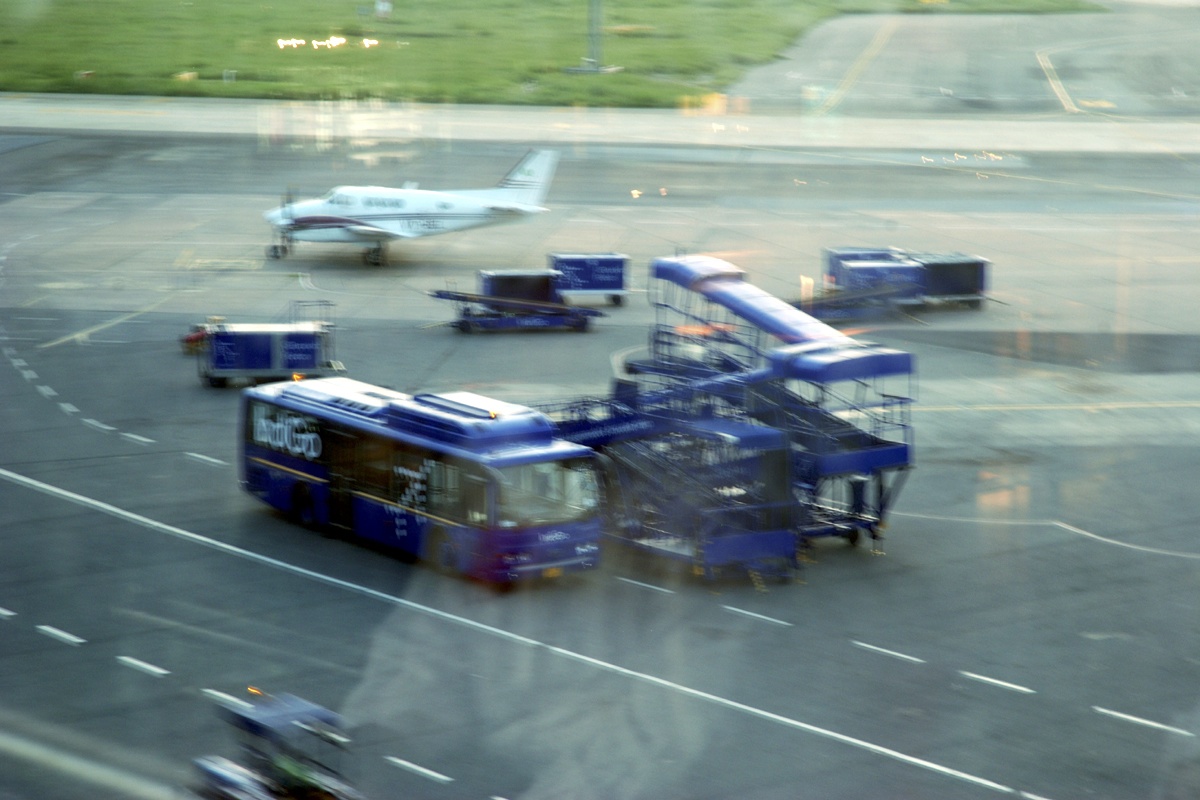The photograph captures a bustling airport runway area on a somewhat shiny, recently rained-on, grey pavement marked with white dashed lines. In the center is a blue bus, branded with what appears to be "B-O-G-R," though the text is difficult to decipher due to the blur. The bus is stationed next to mobile airplane boarding ramps on wheels. Adjacent to them appears to be a baggage handling truck, a small van, and several cargo boxes or containers. In the backdrop stands a small white single-engine airplane with a red stripe, positioned to the left-upper section of the image. The overall scene is viewed through a reflective window, likely from an indoor waiting area, with a faint reflection of a person visible. Beyond the runway is a green grassy field, adding contrast to the industrial feel of the airport operations depicted.